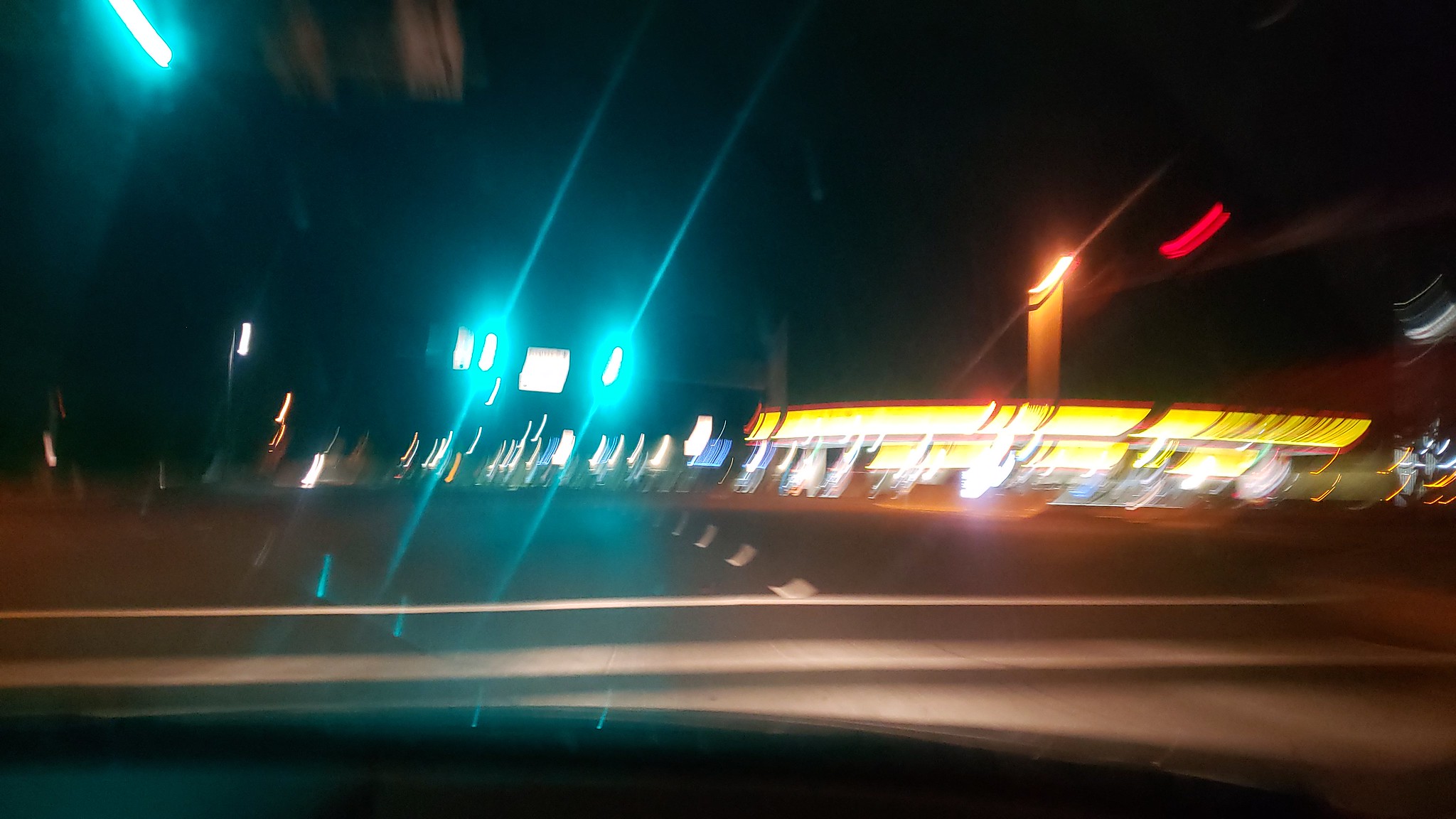This rectangular image captures a blurred, nighttime scene of a road, likely photographed through a car windshield. The disorienting, double-vision effect lends a dizzying quality to the image, with white lines marking the center of the paved road. In the upper right corner, a brightly lit building can be seen, its colors and shape suggesting it is a Waffle House breakfast restaurant, though the words are indecipherable due to the blur. Additionally, several street lights add to the visual confusion, their bright and blinding illumination scattered across the image.